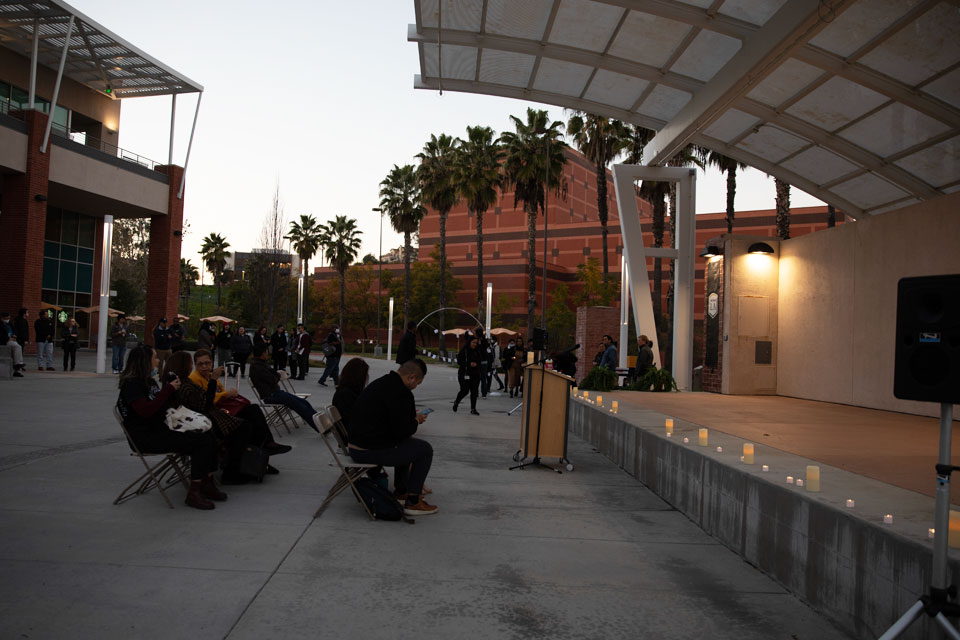This color photo captures an outdoor event, possibly a candlelight vigil, set in a public area that could be in the Middle East or India. The scene features rows of folding chairs, with about six or seven people seated, some talking to each other or looking at their phones, all facing a stage. The stage is adorned with both large and small lit candles and is equipped with a lectern or podium, indicating that someone is expected to speak. In the background, you can see a long rectangular red brick building topped with a smaller structure, along with a line of palm trees. Another large building is also visible in the distance, reinforcing the impression of a campus or park setting. The image seems to be a casual snapshot, capturing the setting and the anticipation of an upcoming event.